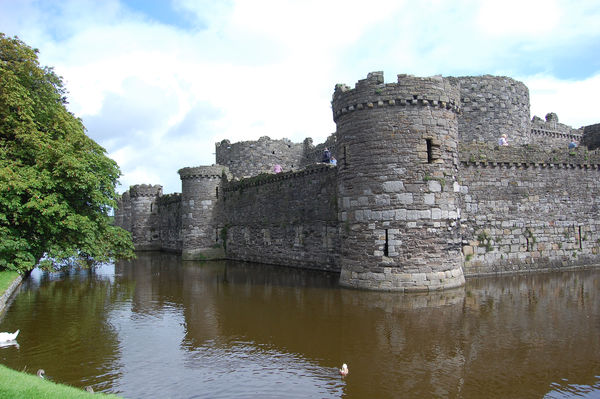This rectangular photograph captures an intricately detailed, large stone castle with a moat, viewed from the near edge of the water. The image features a prominent tree with lush green leaves on the left side, partially overhanging the moat, with patches of green grass visible at the lower left corner and along the left edge. The castle, made of gray stone, has numerous rounded towers positioned at the corners and midsections, creating a mix of rounded and flat, square elements. Moss or small plants grow between some of the bricks, adding a touch of nature to the stonework. The muddy brown moat, with occasional reflective patches of lighter gray from the sky, encircles the castle. A few white ducks are floating on the water's surface. The sky above shows a variety of hues, ranging from light blue to greenish, with a mix of fluffy white clouds providing a picturesque backdrop. Sightseers can be spotted on the castle’s upper level, enjoying the expansive view.